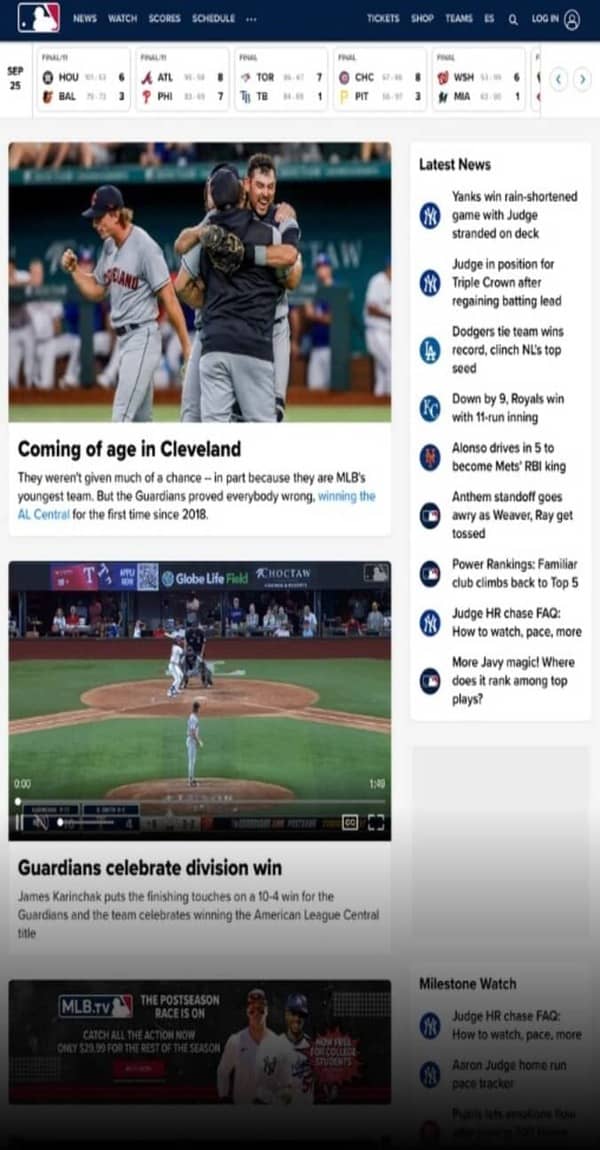A detailed caption for the image is:

"This image appears to be a screenshot from a mobile phone, displaying the main page of a baseball app or website. Dominating the top of the page is a blue navigation bar featuring the baseball logo and various menu options such as News, Watch, Scores, Tickets, and Login. Directly below this bar, there is a section showcasing recent game results, with the winning teams listed above the losing teams.

Beneath the game scores, the page displays three prominent news articles accompanied by images. The first image shows three men embracing while another man walks away, with the headline 'Coming of Age in Cleveland.' The second image captures an action shot from a game, titled 'Guardians Celebrate Division Win.' The third image and article are not described, but they follow the same thematic elements of baseball news coverage.

Running along the right side of the screen, there's a white sidebar labeled 'Latest News,' featuring approximately eight additional clickable articles. At the bottom of the page, a section marked 'Milestone Watch' is present, indicating notable achievements and records within the sport. The overall layout is clean and designed for easy navigation, catering to avid baseball fans looking for the latest updates and scores."